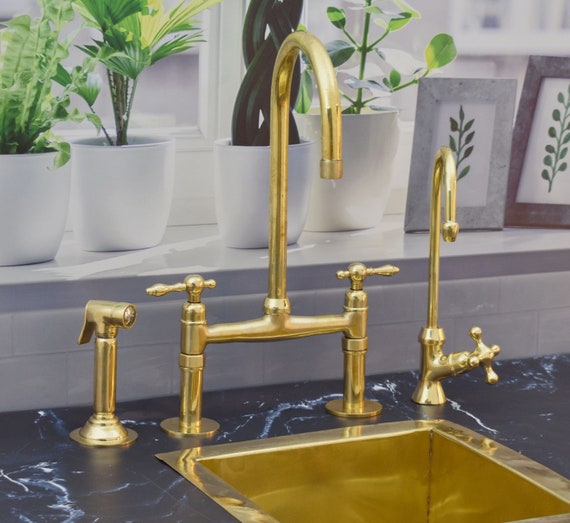The photograph captures an elegant kitchen countertop, spotlighting a luxurious, bright gold sink ensemble set against a sleek black marble countertop with white streaks. The sink itself is square with three distinct water dispensers. On the left, there is an extendable sprayer handle for pressure washing. At the center, the main faucet features a prominent, cane-like curved design, flanked by hot and cold knobs. On the far right, a smaller, dedicated hot water dispenser mirrors the graceful curves of the larger faucet. 

Behind the striking gold appliances is a white tiled backsplash leading to a gray windowsill which houses a vivid array of green plants. Each of the four distinct plants is potted in identical white ceramic vases, bringing a touch of nature into the space. To the right of these living decorations, two minimalist framed artworks showcase delicate plant stems and leaves, adding an artistic accent to this sophisticated kitchen scene.